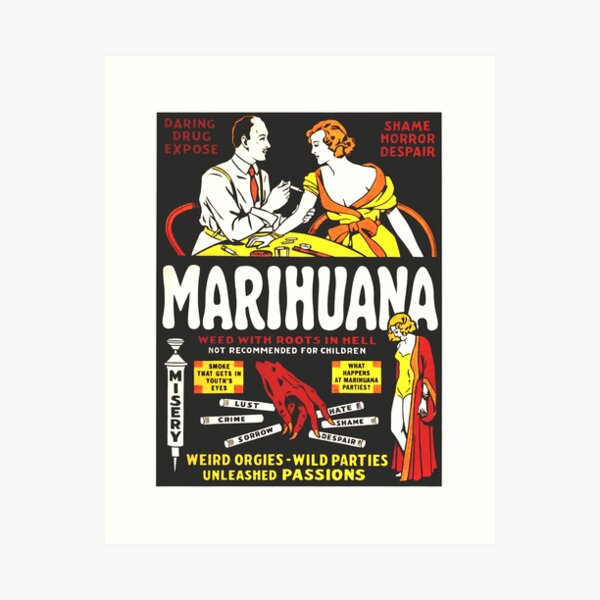In this vintage-style advertisement, starkly set against a black background, bold red letters at the top left proclaim "Daring Drugs Exposed," while the top right screams "Shame, Horror, Despair." Dominating the center is an image of a man on the left side, appearing to inject a woman on the right side, who has orange hair and is dressed in an orange robe over a yellow dress. The table in front of them is cluttered with various objects, adding to the chaotic and desperate atmosphere. Below the central image, large, ominous text reads "Marahuana" with a sensational subtitle, "Weed with Roots in Hell Not Recommended for Children." 

At the bottom of the ad, a sinister red, claw-like hand—suggestive of the devil—grasps at words like "Misery," "Lust," "Crime," "Sorrow," "Hate," "Shame," and "Despair," which are scrawled around it, emphasizing the ad’s dramatic warning against drug use. The lower part of the poster also vividly describes the consequences of drug use with phrases like "Weird Orgies," "Wild Parties," and "Unleashed Passions" laid out in yellow text. The advertisement clearly aims to deter drug use through a mix of fear and moral condemnation, using vivid imagery and stark contrast between red, white, and yellow fonts against the black background to heighten its impact.